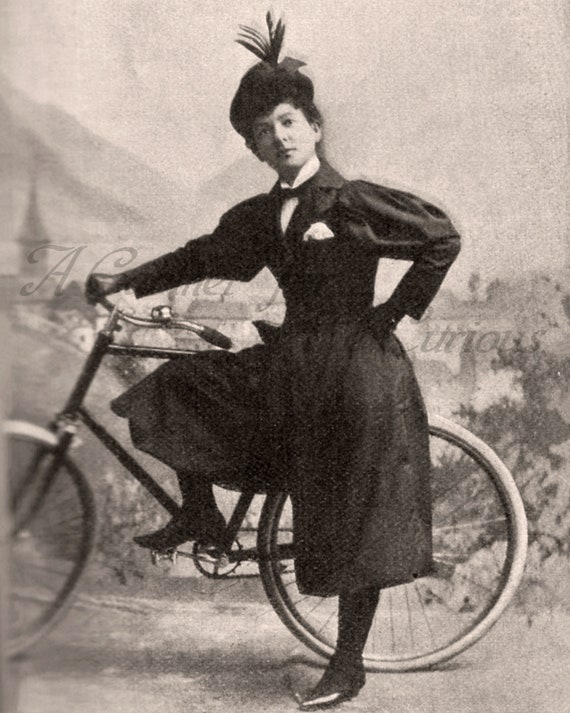This is a sepia-toned vintage photograph possibly from the late 1800s or early 1900s, depicting a woman confidently standing beside her bicycle. The woman has light skin and is dressed in a formal, black Victorian-style ensemble featuring a long dress with frilled shoulders, long sleeves, and a white undershirt with a slight collar peeking out. She is also wearing pointed, short-heeled shoes with black socks. Her left hand rests on her hip while her right hand grasps the steel handlebars of the bicycle, and she strikes a poised stance with her right foot on a pedal and her left foot grounded. The woman's outfit is topped with a black hat adorned with striking black feathers that shoot out from the center. Her facial expression is serious, and she gazes directly at the camera with an air of confidence.

The bicycle beside her, with its large white wheels and prominent spokes, has a black frame and curved handlebars. The blurry background, suggesting an outdoor setting, features some foliage on either side, a line of buildings including one with a steeple, and the faint silhouette of mountains possibly indicating a village's outskirts. There is also some unreadable text or watermark present in the photo, suggesting it may have been digitally altered or marked by an archive. The overall image exudes a nostalgic aura, capturing a moment of poised elegance in a historical context.